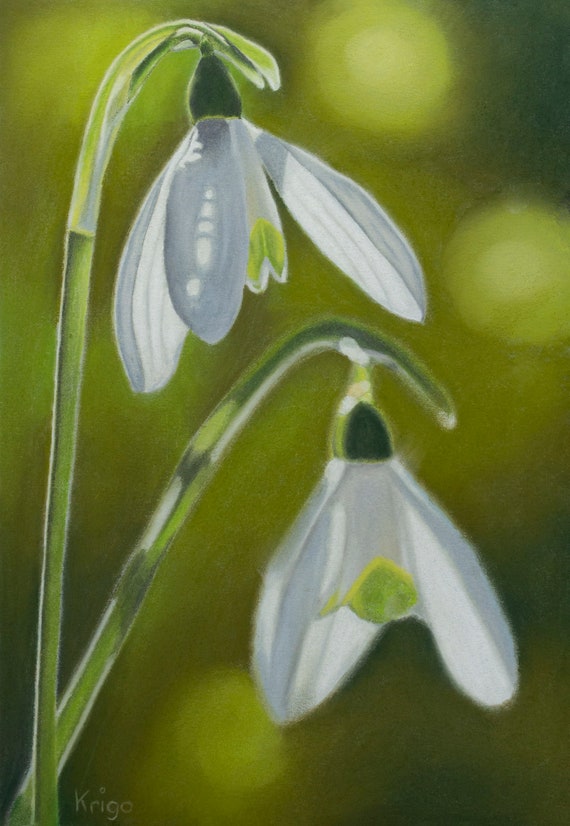This image, seemingly a painting, showcases two prominent white-petaled flowers with green stems against a blurred, watercolor-like background in shades of green, grey, and black. Strokes of a brush suggest it might be an acrylic, oil, or gouache painting and lend a soft, painterly texture to the image. The first flower's stem originates from the bottom left corner and extends vertically to the top left, where it curves over, allowing the flower to hang downward with its petals pointing down. The second stem also begins at the bottom left but stretches at an angle, moving upwards and curving to the right, mirroring the first flower's hanging posture. Both flowers have delicate white petals and a tiny green interior. Subtle highlights and shading enhance their realistic appearance, while the name "Kringo" at the bottom suggests the artist's signature. The background, appearing almost abstract, features lighter green circles with a hint of yellow, adding depth and a dreamy quality to the scene.